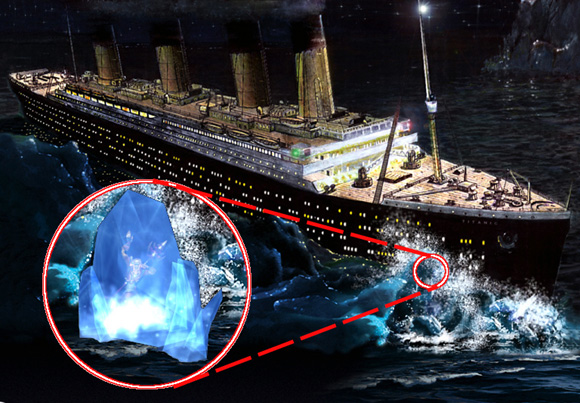The image is a detailed depiction of the Titanic moments before it hits an iceberg. The large, dark-colored ship is illuminated by tiny yellow and white lights emanating from the passengers' cabins. Four prominent smokestacks tower above the upper deck, with one emitting steam. The ship appears to be navigating through rough, dark waters under the night sky. A vertical pole near the front of the ship has a small light attached to it. In the lower right corner of the image, there's a large circle highlighting a close-up of the iceberg, with lines indicating its position in the water in relation to the Titanic. The ship is shown moving towards the right of the picture, directly towards this looming iceberg. The upper deck is sparsely populated, with visible lifeboats, and no people are seen on it. The overall scene captures the eerie and tense atmosphere of the approaching disaster.